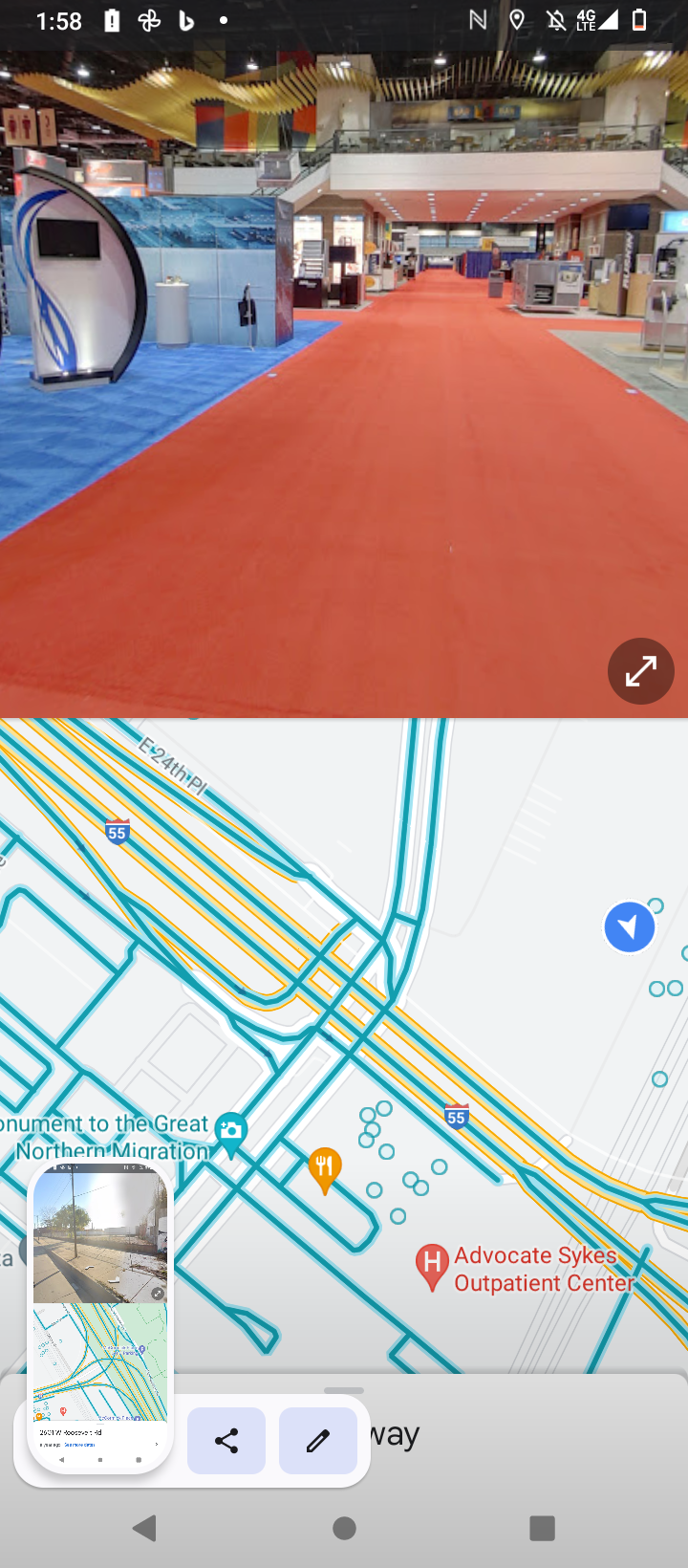The image consists of two stacked rectangular photos, both in a portrait orientation, though not significantly taller than they are wide.

The top photo showcases a long red carpet that extends from the foreground to the background, gradually narrowing as it reaches the depth of the image. On the left side, there's a floor area with a blue hue, featuring a white display object against a background of blue tiles with a wavy top border. To the image's right, there is a hint of green flooring and an indistinguishable object, seemingly distant. In the background, a second level with a balcony is visible, characterized by a white facade and glass railing, allowing people to overlook the area below. Additionally, white-yellow wavy elements hang from the ceiling, adding an artistic touch. It appears this photo was taken with a mobile phone, judging by the composition and focus.

The bottom photo is a screenshot from Google Maps, depicting the location pertinent to the above scene. The map is marked by numerous thin teal lines representing roads, intersected by yellow lines denoting a highway, identified as Highway 66. In the upper right-hand corner, a blue navigation arrow is present. The map also features red text labeling "Advocate Skies Outpatient Center," hinting at the location's significance.